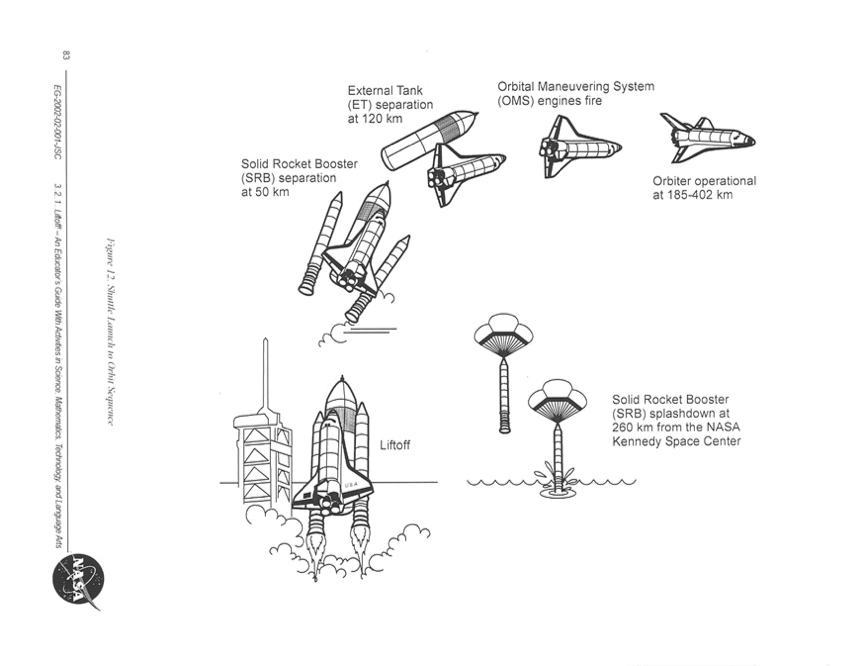This detailed diagram depicts the launch sequence of a space shuttle, accentuating the key stages of its trajectory. Starting at the bottom left of the diagram, the space shuttle's liftoff stage is illustrated, showcasing the shuttle attached to two striped solid rocket boosters (SRBs) and a large central external tank as they ascend into the sky. Moving clockwise, the next stage highlights the SRB separation at an altitude of 50 kilometers, where the two boosters detach from the central rocket. 

The subsequent image demonstrates the separation of the central external tank occurring at 120 kilometers, allowing the space shuttle to continue its ascent independently. Following this, the diagram shows the firing of the Orbital Maneuvering System (OMS) engines, which are essential for adjusting the shuttle's trajectory and achieving orbit.

In the subsequent stage, the shuttle is shown operating in orbit at altitudes ranging from 185 to 402 kilometers. Finally, the diagram illustrates the splashdown of the SRBs at a distance of 260 kilometers from the NASA Kennedy Space Center, with one booster already in the water and the other descending under parachutes. Notably, a thin black line flanks the left side of the image, interspersed with descriptive annotations and positioning the iconic NASA emblem at the bottom.